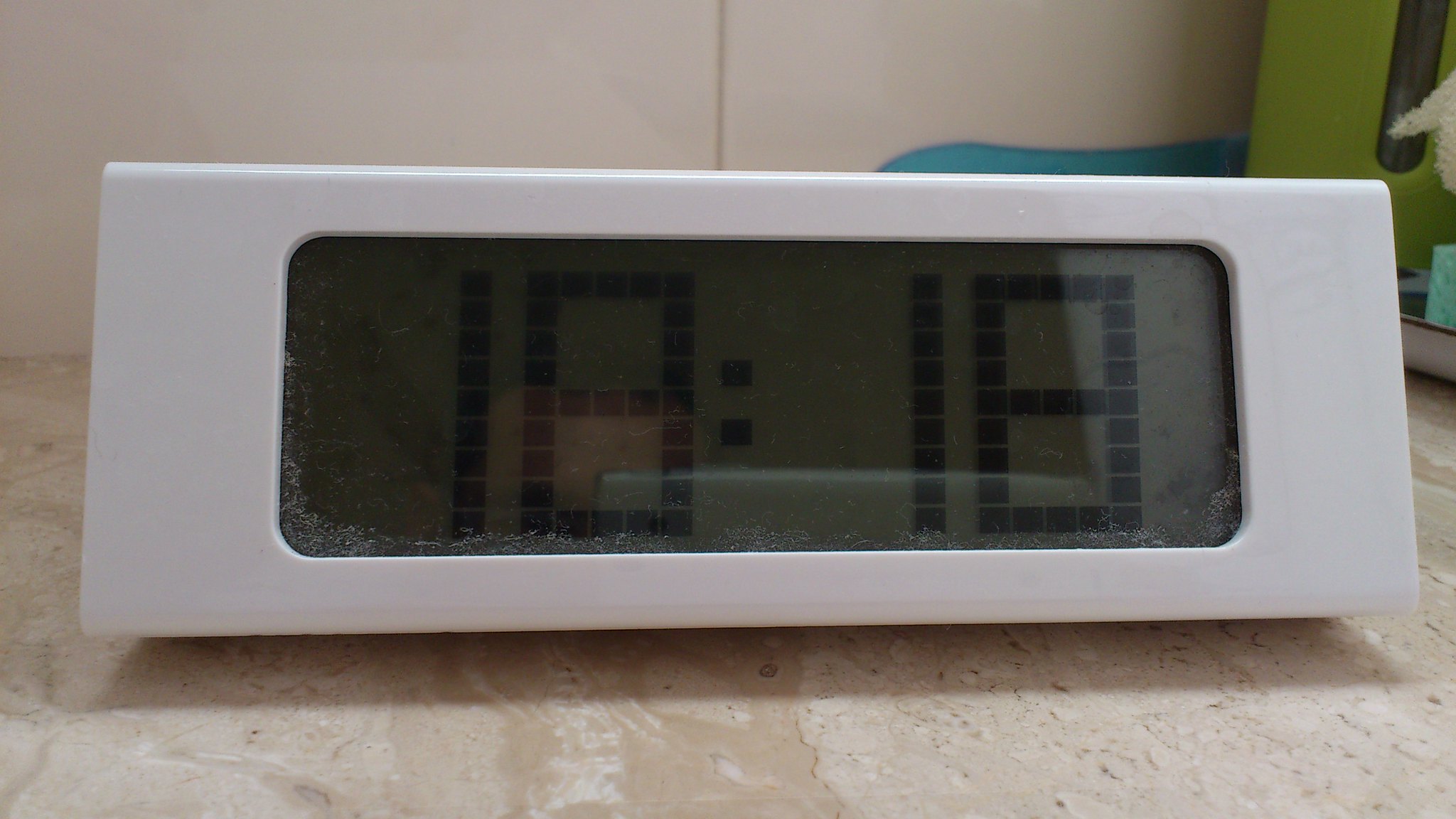This interior photo captures a nostalgic 1970s vibe with a brownish-pinkish marbled countertop as its focal point. In the background, a white paneled wall is visible, its panels marked by a discernible line. A small, rectangular digital clock with a white frame sits prominently in the foreground, displaying the time "18:18." The bottom edge of the clock’s glass is dust-laden, hinting at its age and the room's possibly infrequent use. The background gently fades into obscurity, with a few indistinct objects clustered in the back right, adding an air of mystery to the setting.